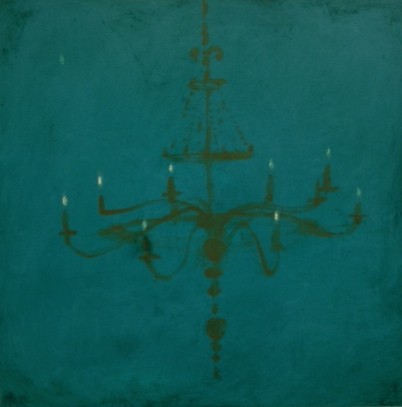The image depicts a murky and abstract painting of a vintage chandelier, likely from the early 1900s, with a predominantly dark seafoam or blue-green background that fades to blackish shadows at the corners. The chandelier, though faded and shadowy, features eight long, looping black arms, each holding what appears to be a lit candle, casting a soft white glow. The chandelier is adorned with cylindrical ornamental balls hanging from its bottom center and additional elaborate ornaments resembling a beaded lampshade near the top. The overall impression is one of quiet reflection, captured through the painting's soft, cloudy aesthetics, giving it an air of introspective tranquility.